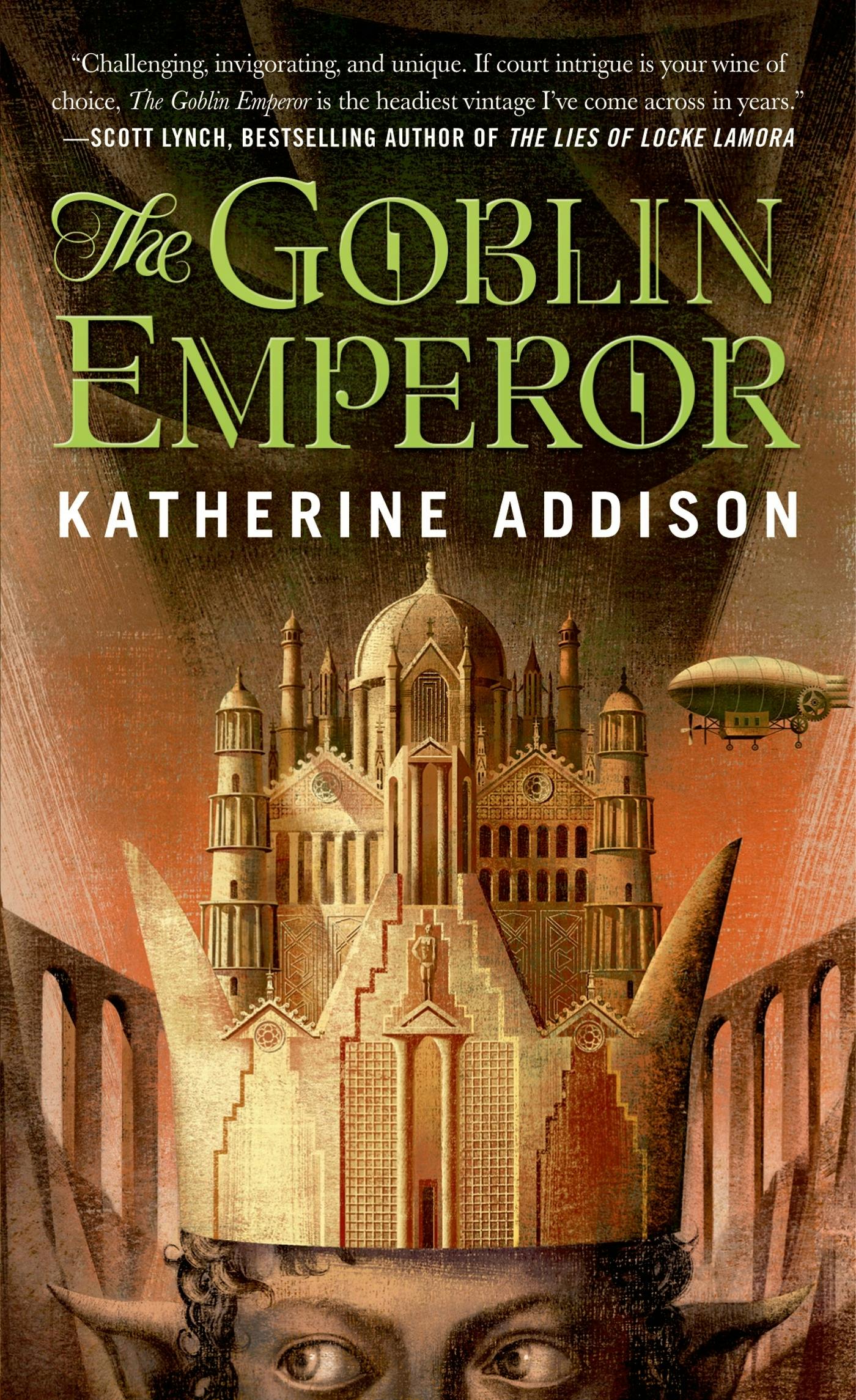The cover of the book, "The Goblin Emperor," by Catherine Addison features a striking and surreal illustration. Dominating the cover is an image of a person—possibly representing an elf or a goblin—who gazes off to the left. The figure wears an elaborate golden crown that intriguingly resembles a grand architectural structure with domes and columns, evoking comparisons to the Taj Mahal and other temples. Additionally, a zeppelin or blimp gracefully floats across the top right of the scene, adding to the whimsical yet regal atmosphere.

Above the artwork, a quote in white text attributes high praise for the book: "Challenging, invigorating, and unique. If court intrigue is your wine of choice, The Goblin Emperor is the headiest vintage I've come across in years," by Scott Lynch, bestselling author of "The Lies of Locke Lamora." Prominent green text spells out the title, "The Goblin Emperor," while the author's name, "Katherine Addison," appears below in bold, white, all-capital letters. The vibrant and imaginative artwork, combined with glowing reviews, makes for a compelling and unique book cover.